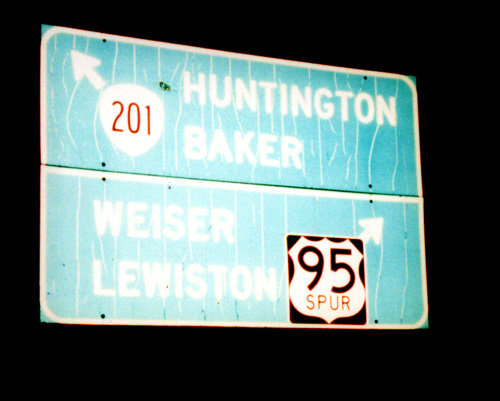This image captures a weathered green highway sign, photographed at night with a flash, accentuating its reflective surface against a pitch-black background. The sign has two distinct sections. The top half directs drivers to "Huntington Baker" with a black Route 201 symbol and a left-pointing arrow. Beneath, the lower half instructs on directions to "Wiesen" and "Lewistown," featuring a white Interstate 95 shield with the text "SPUR" inside a black box, accompanied by a right-pointing arrow. Both sets of destinations—Huntington Baker, Wiesen, and Lewistown—are marked with white text. The sign shows significant wear, suggesting long-term use or possible storage after replacement.